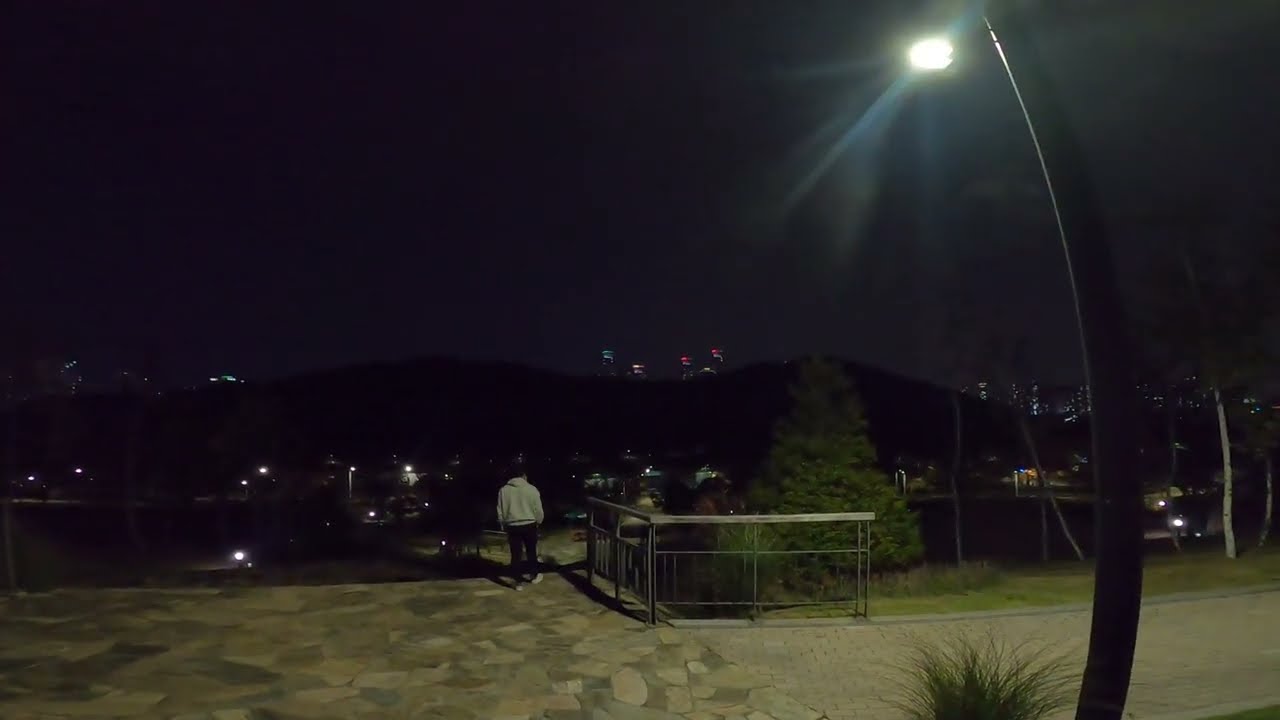The nighttime image depicts an outdoor scene with a man in a gray hoodie, dark pants, and white tennis shoes standing at the center. He is positioned on a cobblestone path, which transitions into a tan brick walkway to his right. The man's back faces us as he gazes into the dimly lit expanse. To the right of the man is a curved light pole illuminating the immediate area, and nearby is a green bush. Behind him is a small fenced area with a large tree, and additional greenery includes more trees in the foreground. Beyond this area, the image reveals the silhouettes of rolling hills, scattered buildings, and various colored lights—including red, blue, and white—dotting the landscape. The background grows progressively darker, with hints of skyscrapers and street lights illuminating the distant nighttime skyline.